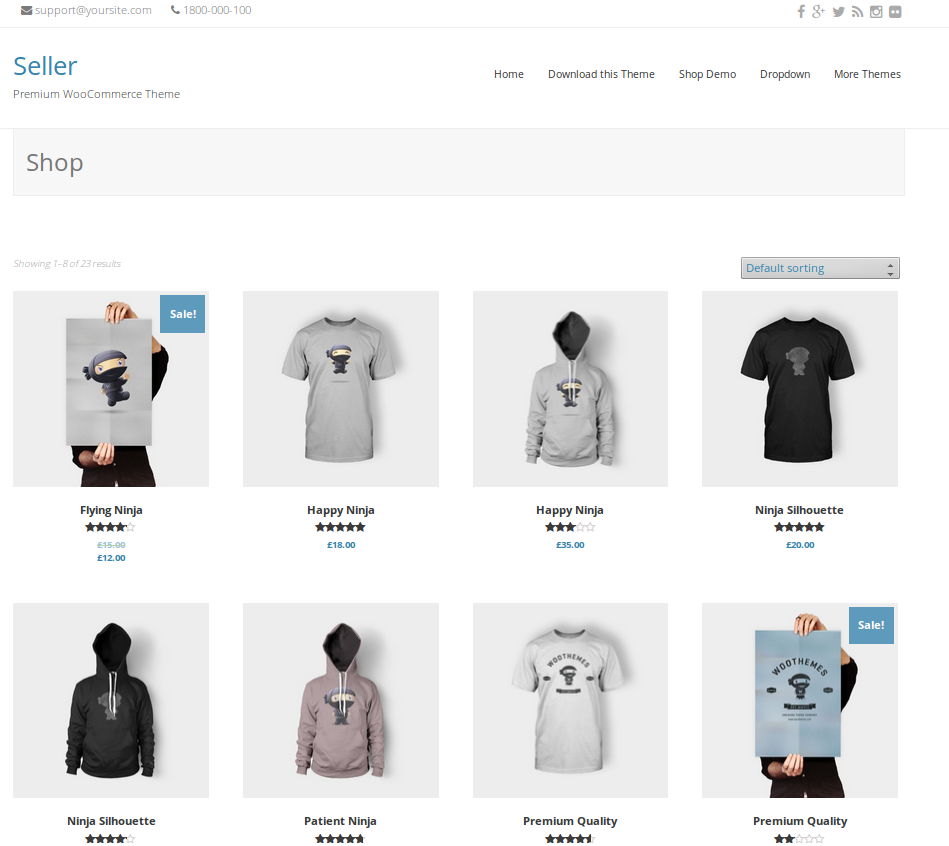This image is a screenshot taken in portrait mode from a shopping website. The arrangement showcases various site elements and a selection of apparel products, providing a template for creating an e-commerce platform.

At the top of the screen, the header, set against a white background, prominently features the word "Shop" in a gray stripe. Above this, a blue stripe displays the website's title, "Seller," along with a subtitle, "Premium WooCommerce." In the upper right corner, navigation headers include "Home," "Download this Theme," "Shop Demo," and a dropdown menu titled "More Themes." The upper left-hand corner displays contact information placeholders: "email support@your site.com" and "Phone," while the upper right includes social media icons for Facebook, Google+, Twitter, and Instagram, suggesting connectivity and interactivity options.

Further down, the image's main content area consists of a product grid sorted from one through eight out of a total of 23 results. This sorting information appears on the left side of the page, while a blue menu on the right side indicates "Default Sorting," which determines the order of the displayed items. 

The bottom two rows of content highlight various types of t-shirts and hoodies. Each product image includes an overlay of the product name, its star rating, and, in most cases, the price. However, in this particular image, the price for the bottom row of products is not shown, suggesting a partially scrolled page view, emphasizing the interactive nature of the design.

This screenshot is a template meant for individuals creating their own website, offering a structured layout that includes clear navigational aids, social media integration, and a methodical product display for potential e-commerce ventures.